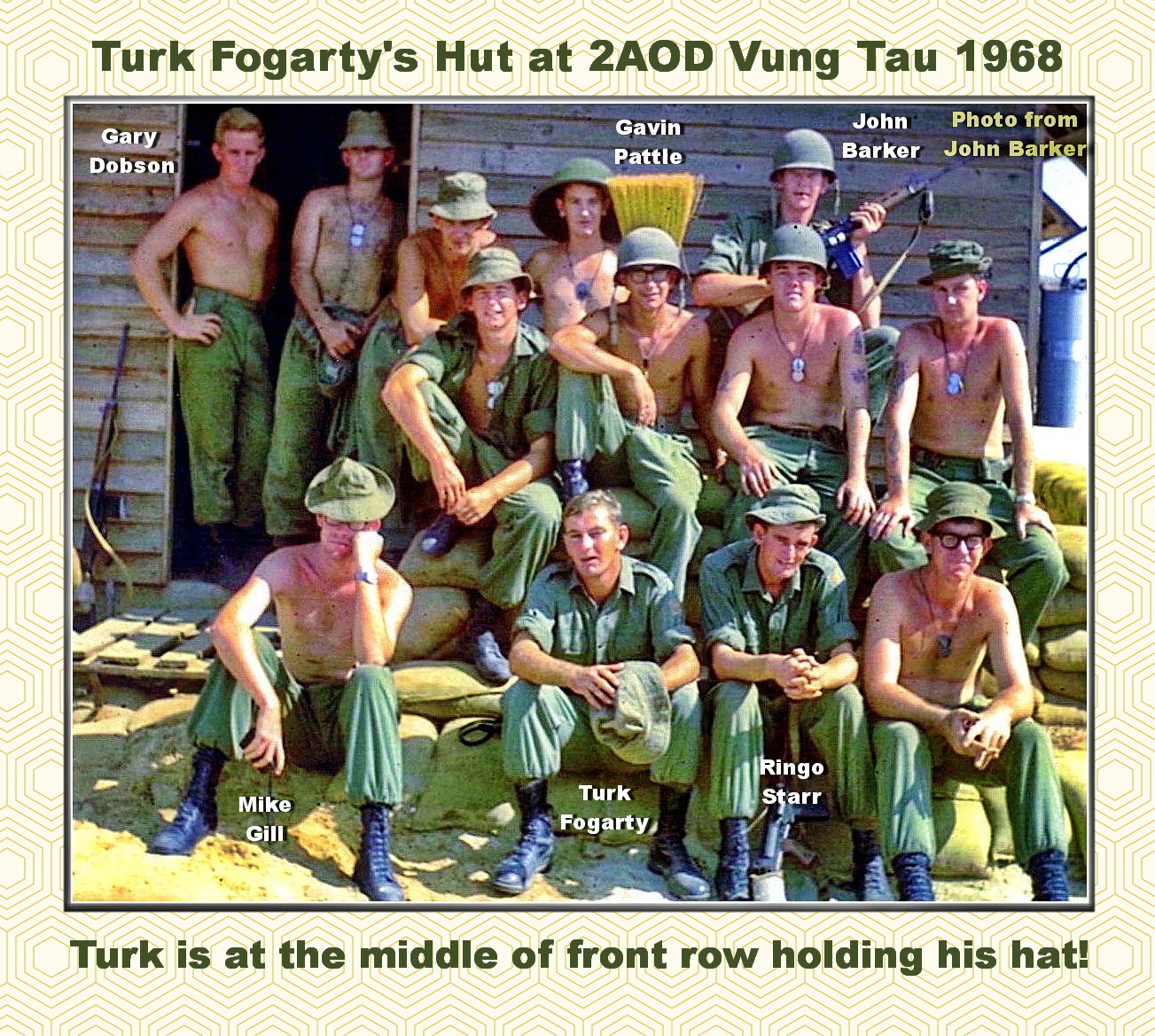This photograph, taken in 1968, captures a group of soldiers during the Vietnam War, posed in front of a wooden barracks labeled as "Turk Fogarty's Hut at 2 AOD, Vung Tau." The image features an irregular pentagonal pattern, likely computer-generated, framing the scene. The soldiers, many of whom are shirtless, are arranged in three rows: a back row standing, a middle row seated on a pile of sacks, and a front row closer to the ground. Notably, Turk Fogarty is identified standing in the middle of the front row, holding his hat, as indicated by the white text below the image. Other named individuals include Gary Dobson, Gavin Patty, John Barker (top right), Mike Gill, and Ringo Starr, with John Barker’s name highlighted in yellow. The clear outdoor setting, coupled with the visible details and names, emphasizes the camaraderie and environment of these soldiers during a significant historical period.